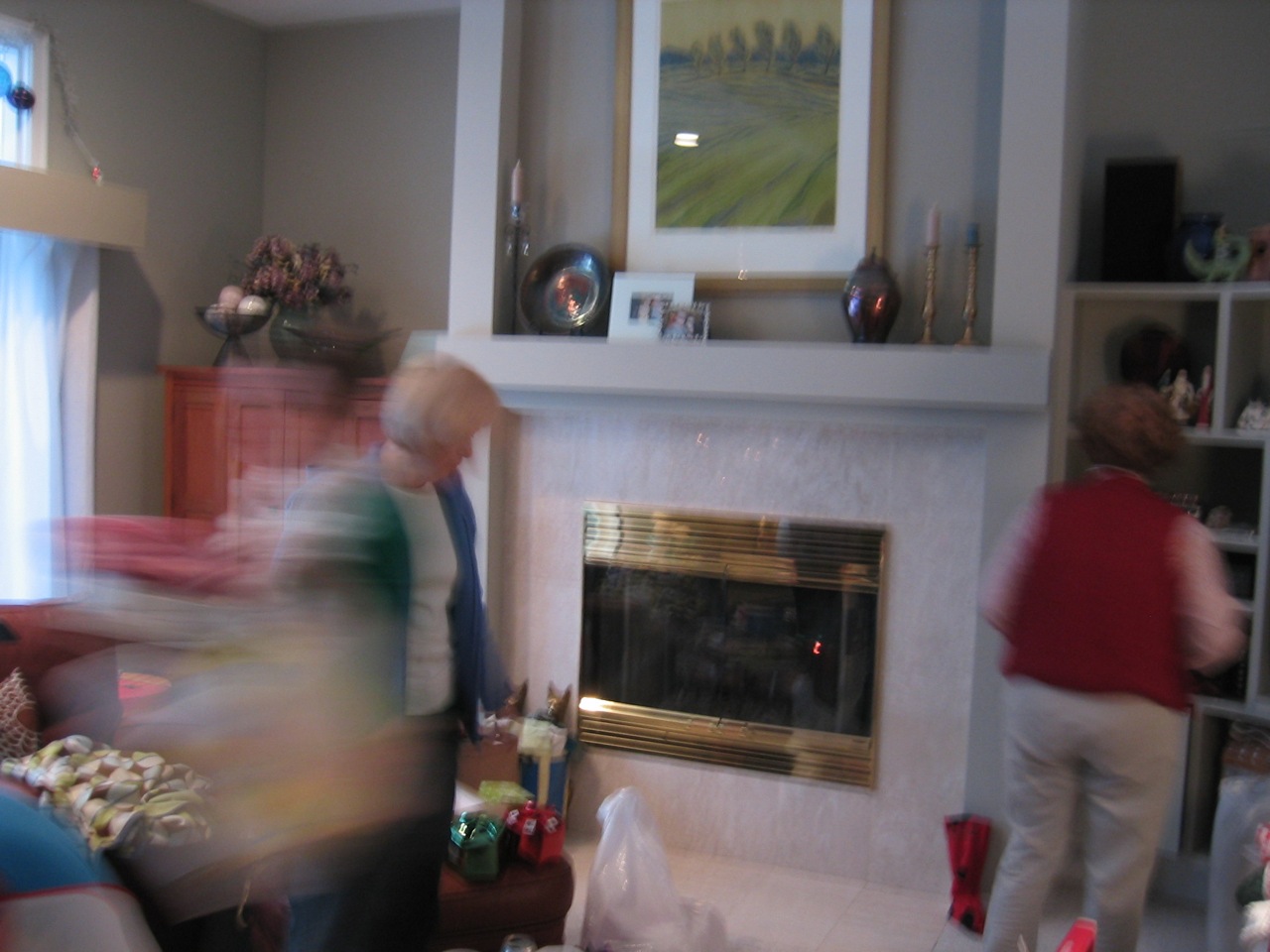The image is a somewhat blurry color photograph taken indoors, capturing a living room, possibly during a celebration such as Christmas. In this cozy living space, the focal point is a fireplace located on the far wall. The fireplace features a glass front with gold or brass-colored borders and a white mantel adorned with a small decoration. Above the mantel hangs a piece of artwork in a wooden frame. The room is lit festively with a string of red fairy lights around a window frame on the left side of the image, suggesting a holiday atmosphere. In front of a dark brown leather sofa, which has two small wrapped gifts in shiny red and green paper on its edge, sits a large plastic bag on the floor to the right.

In the living room, two women are captured in the frame. The woman on the right, seen from behind, has white hair and is wearing a blue cardigan over a white t-shirt. She appears heavyset and is engaging with the room. The other woman, on the left, is blurred due to movement during the photograph. She has brown hair, wears a sleeveless red shirt and khaki pants, and stands facing the white shelves. The walls of the room are a light gray, completing the warm and inviting holiday scene.